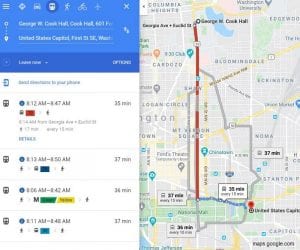This image displays a Google Maps navigation page with detailed directions from George Cook Hall to the United States Capitol in Washington, D.C. The image shows four different transit options, each row providing a specific set of times and estimated travel durations. Here’s a breakdown of the rows:

1. **First Row**: Departure time from 8:12 to 8:47 a.m., with an estimated travel time of 35 minutes, presumably on the Red Line.
2. **Second Row**: Departure time from 8:13 to 8:50 a.m., with an estimated travel time of 37 minutes, presumably on the Blue Line.
3. **Third Row**: Departure time from 8:06 to 8:42 a.m., with an estimated travel time of 34 minutes, presumably on the Green and Yellow Lines.
4. **Fourth Row**: Departure time from 8:11 to 8:48 a.m., with an estimated travel time of 34 minutes, presumably on the Light Blue Line.

Each row features a blue clock icon with the times clearly indicated. The leftmost column shows symbols suggesting that the routes are by metro train, and the second row beneath the times likely indicates the line colors. 

To the right half of the page, the map prominently features a red vertical line connecting the two destinations. This line illustrates the primary route, which includes walking segments marked by blue dotted lines common in Google Maps. Four pop-up boxes along the route highlight the timing details for each transit option. Additionally, gray lines indicate less direct alternate routes that appear less straight.

At the bottom left of the map, a gray box notes "Maps by Google." The background largely features urban streets with major roads highlighted in yellow and smaller roads in white. A park area is seen towards the bottom of the map, further emphasizing the city’s landscape.